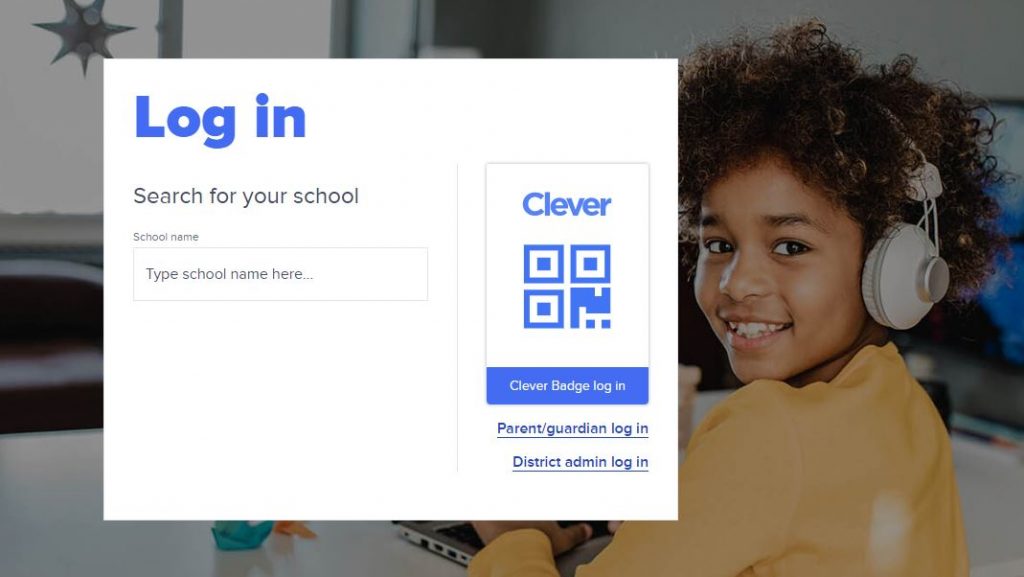The image is a screenshot of the Clever website's login page. The background features a vibrant photograph of a cheerful child wearing headphones, seemingly engaged in an online activity, possibly using a laptop. Although the laptop itself is obscured by the login window, the background suggests a productive and engaging learning environment.

The login window, which occupies the center of the screen, has a clean white background. At the top, there's a prompt that reads, "Search for your school," followed by fields labeled "School Name" and a search bar for users to enter their school's name. To the right of these fields, the Clever logo is prominently displayed, consisting of a grid of what appears to be two by two squares, with the bottom square somewhat jumbled or incomplete. Below the logo, there’s an option labeled "Clever Badge Login."

Further down the login window, two additional options are available: "Parent/Guardian Login" and "District Admin Login," each with their respective links. Adding to the warm and welcoming ambiance of the image, on the left side of the desk near the student, there are two origami shapes, one possibly a blue crane, highlighting a creative and nurturing environment.

In the background of the image, beyond the focal login window and the working child, there are windows that let in natural light, contributing to the scene’s bright and positive atmosphere. Hanging in one of these windows is a star-shaped decoration, adding a whimsical and decorative touch to the learning space.